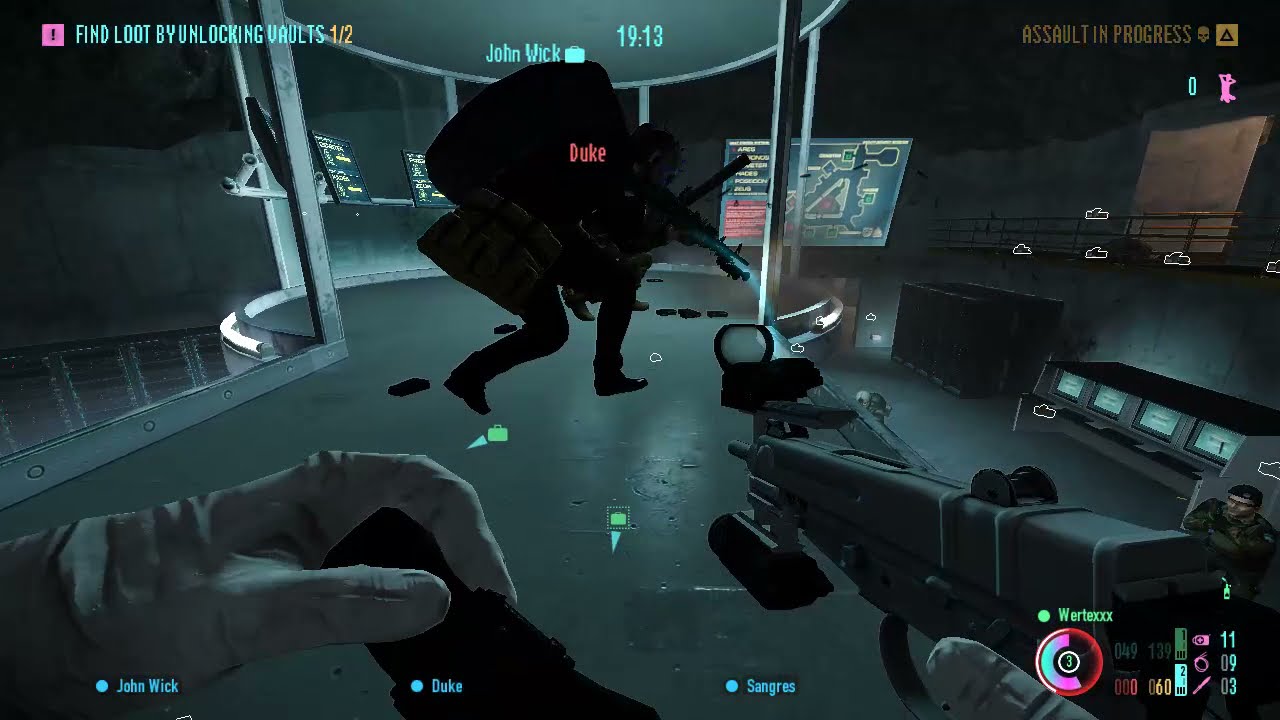The image is a detailed still screenshot from a first-person shooter video game. The scene is set against a dark bluish-gray background and features a horizontal rectangular layout. In the upper left corner, there is a pink square accompanied by white text that reads, "Find Loot by Unlocking Vaults 1-2." Centrally, the main game environment showcases a silhouetted character labeled "John Wick" in light blue text, standing on an illuminated white neon platform. Above John Wick’s name, a timer reads "19:13." 

To the very right, faint gold text over the dark background indicates an "Assault in Progress." The player's perspective is from a first-person view, where the foreground shows gloved hands handling a weapon—a long-barreled gun with a small scope. The right hand is noticeably on the trigger, aimed at John Wick, and the left hand appears to be holding another item, possibly an ammo clip.

At the bottom of the image, names like "John Wick," "Duke," and "Sangris" are listed in small columns. Additionally, a pink and white circle is present here, with unreadable white text above it, emphasizing the multiplayer aspect of the game. The image captures a moment of intense gameplay where the player's actions are crucial to the mission's success.